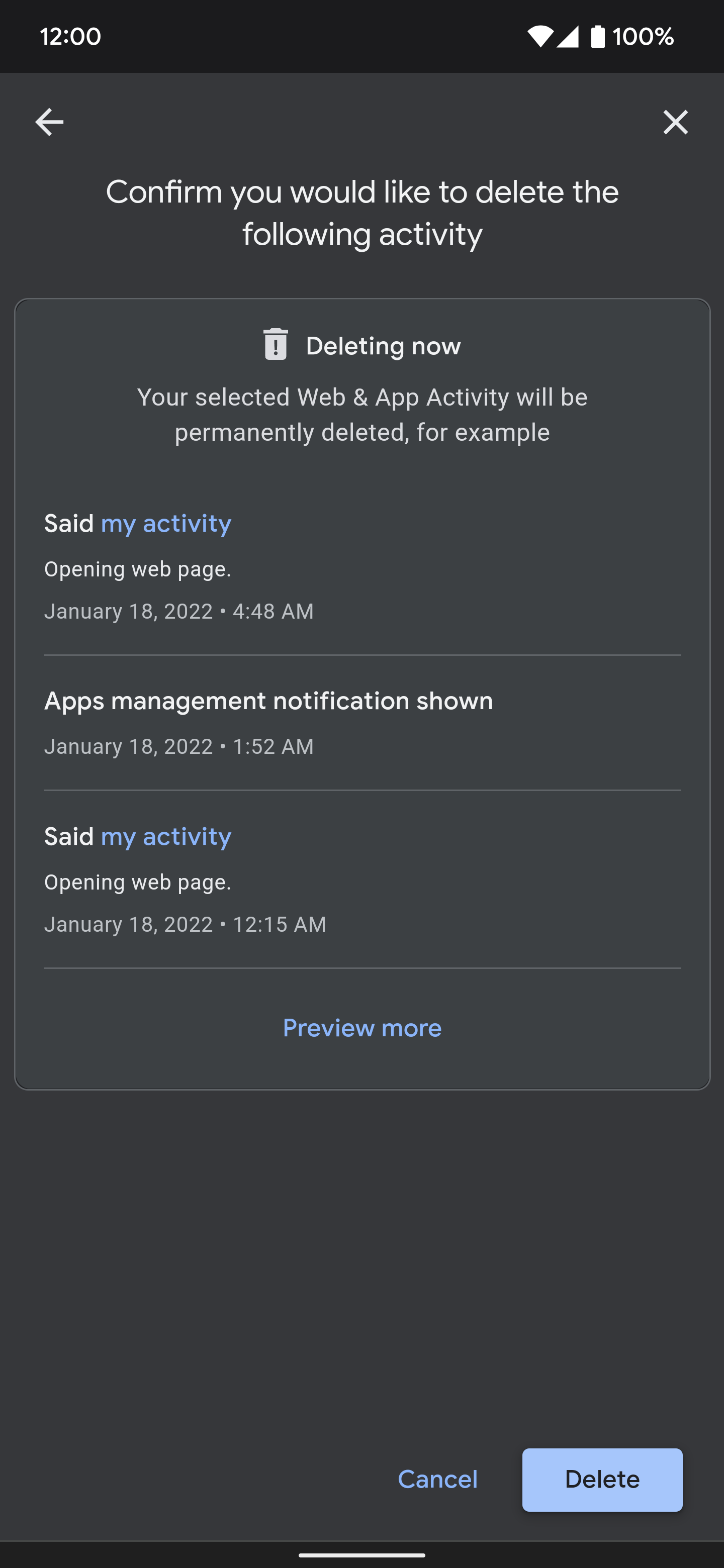This is a detailed screenshot from a smartphone operating system, likely Android or Google, but not Apple. At the very top of the screen is a slim black bar stretching from edge to edge, featuring white text and icons. On the left, it displays the time as "12:00," and on the right, it shows "100%" along with a battery icon, a Wi-Fi icon, and a signal strength icon, all in white.

Directly beneath this, the screen transitions to a dark gray background. At the top left is a left-facing arrow, possibly for navigating back to a previous menu. On the top right, there is an "X" symbol for canceling the current operation.

The main section of the screen displays a prompt in white text asking, "Confirm you would like to delete the following activity." Below this prompt is a lighter gray bar with a trash can icon, along with text stating "Deleting now." It further specifies, "Your selected web and app activity will be permanently deleted, for example."

Beneath this, there are three short paragraphs detailing specific activities such as "Identifying activity," "Apps management notification," and "My activity opening a web page."

Towards the bottom of the screen, there is a blue hyperlink text that says "Preview more." Finally, at the bottom right-hand corner, there are two toggle buttons: a gray "Cancel" button, and a light blue "Delete" button with black letters.

This screenshot provides a comprehensive view of a deletion confirmation dialog within the smartphone's operating system.